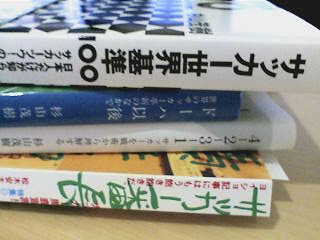This photograph features a stack of four books resting horizontally on a light-colored, shiny wooden table. The books are written in an Asian language, although their exact titles remain unreadable due to the oriental characters. From top to bottom, the first book has black text on a white cover. Below it, the second book features white text on a blue cover. The third book is white with black text and displays the numbers "4-2-8-1" in a vertical orientation along the spine. The bottom book has a white spine adorned with green, red, and blue text, and a multicolored brown design on the top. The stack of books occupies most of the frame, emphasizing their distinct colors and arrangement.